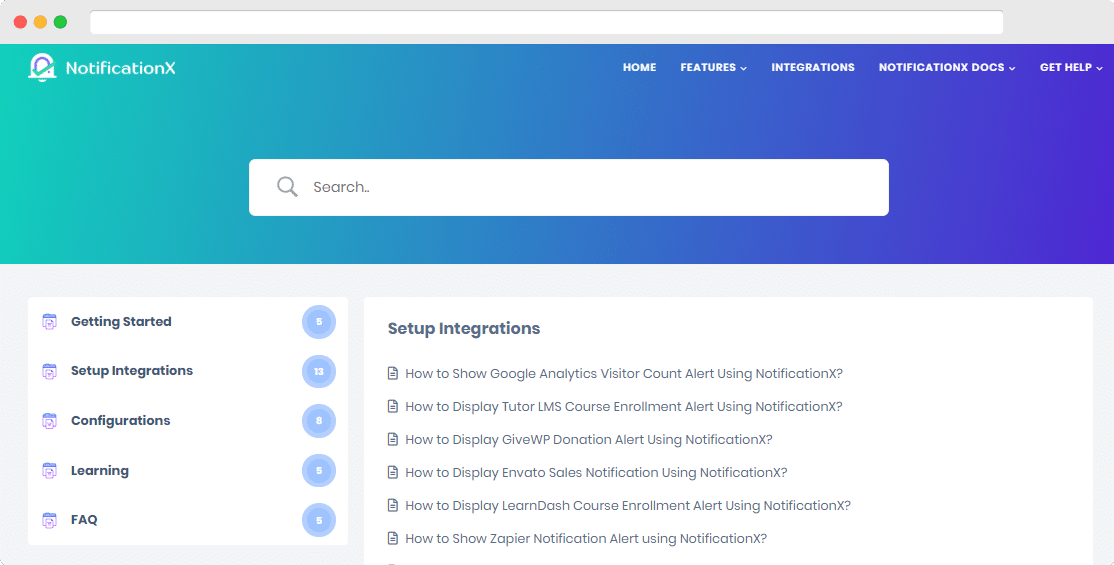This web page for "NotificationX" features a clean, intuitive layout, starting with the browser's top bar containing three horizontally aligned buttons: a red close button, a yellow minimize button, and a green maximize button. Beneath this, there is a combined search and address bar. The page itself boasts a vibrant banner that transitions from teal to purple. 

Under the banner, there are five horizontal navigation tabs: "Home," "Features" (with a dropdown menu), "Integrations," "NotificationX Docs" (with a dropdown menu), and "Get Help" (with a dropdown menu). Next to these tabs is a white search bar.

The main content section below contains a vertical sidebar with categories: "Getting Started," "Setup," "Integrations," "Configuration," and "Learning Facts." Alongside this sidebar, the main content area is organized horizontally with guides and tutorials, including:

- How to show Google Analytics visitor count alerts using NotificationX
- How to display Tutor LMS course enrollment alerts using NotificationX
- How to display GiveWP donation alerts using NotificationX
- How to display Envato sales notifications using NotificationX
- How to display LearnDash course enrollment alerts using NotificationX
- How to show Zapier notification alerts using NotificationX

Each guide provides step-by-step instructions for integrating and utilizing NotificationX with various platforms and services.